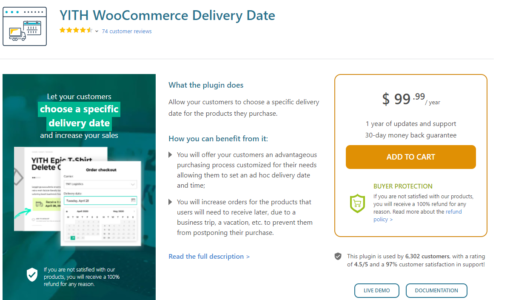The image showcases the **YTH WooCommerce Delivery Date plugin** interface for a popular e-commerce platform. At the top, the title "YTH WooCommerce Delivery Date" is displayed prominently in a bluish-green color, accompanied by a rating of approximately 4.5 stars based on 74 customer reviews. 

Further down the page, there is a detailed description in blue, highlighting the main functionality of the plugin: it allows customers to choose a specific delivery date for their purchases. The description explains the benefits for merchants, emphasizing an enhanced purchasing process tailored to customer needs. It notes the potential for increased orders from users who need flexible delivery times due to business trips or vacations, thereby preventing postponed purchases.

To explore more details, there's a clickable button labeled "Read the Full Description" in blue. To the right side of the page, the pricing information is featured— the plugin costs $99.99 per year, which includes one year of updates and support along with a 30-day money-back guarantee. An orange "Add to Cart" button is prominently displayed beneath this information.

Additionally, the buyer protection policy is outlined, reassuring customers that they will receive a 100% refund if they are not satisfied with the product. A clickable section provides further details on the refund policy. 

At the bottom, the plugin’s popularity is highlighted: it is used by 6,302 customers, boasts a 4.5 out of 5-star rating, and has a 97% customer satisfaction rate in terms of support.

To the left of the text, there's an image illustrating the user interface of the plugin, captioned with "Let your customers choose a delivery date." This image showcases various application features and screenshots of the plugin in action.